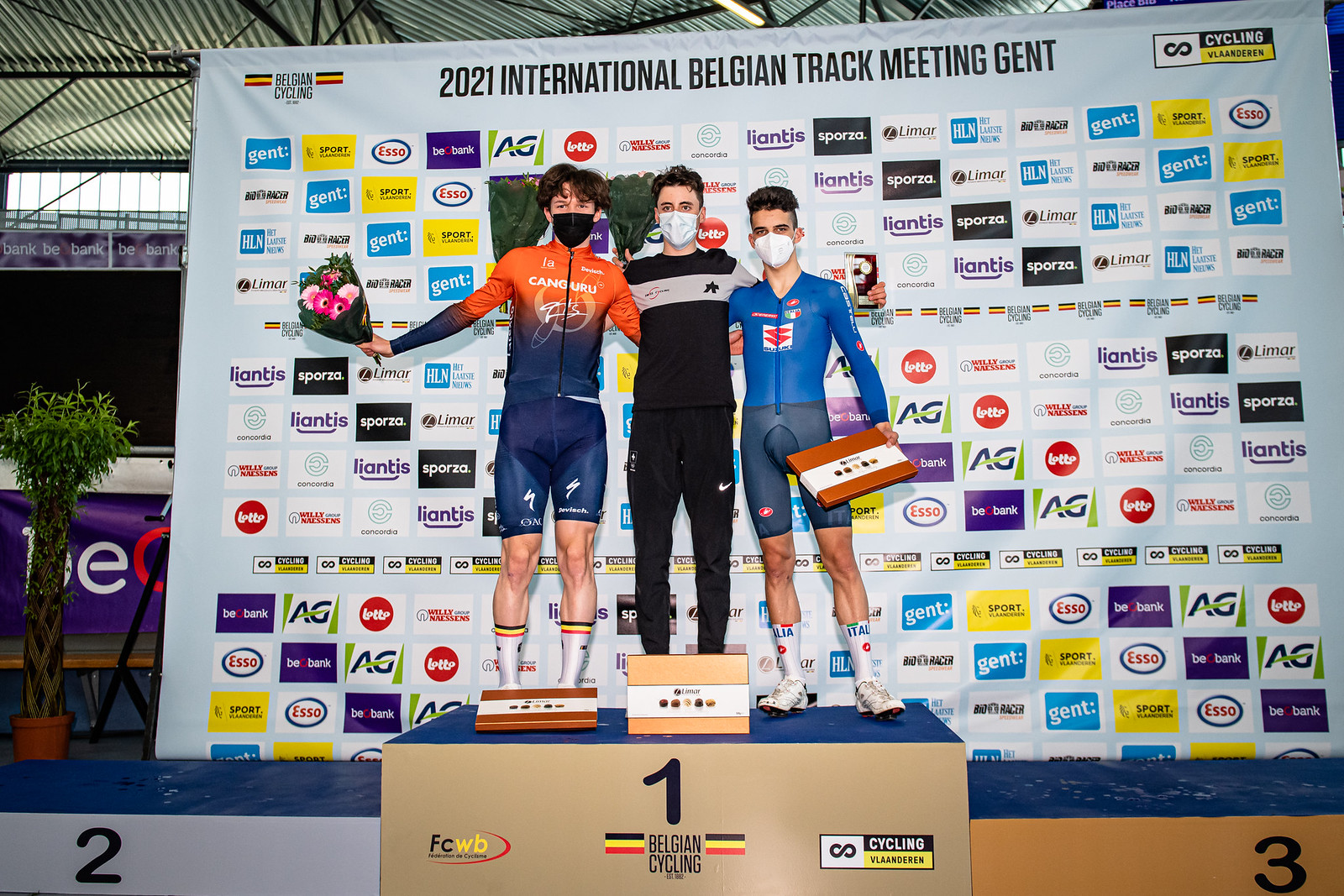In this horizontally aligned rectangular image, three young men are standing on a blue-covered first-place podium during an award presentation at the 2021 International Belgian Track Meeting Gent. The face of the podium step is brown with a black number one in the center, and adjacent lower steps for second and third place are visible. 

All three men, who have short brown hair and are wearing white masks, are positioned centrally in the image. The man on the right is dressed in a tight-fitting blue biking outfit and holds a rectangular box, resembling a box of chocolates with a white label, in his left hand. His right arm is around the man in the middle, who is clad in all black. The man in the middle has both arms around the individuals on either side of him. The man on the left wears an orange and blue top with blue biking shorts, holding a bouquet of flowers in his right hand.

Behind them, a large banner displays the event name, "2021 International Belgian Track Meeting Gent," along with multiple rectangular sponsor logos, including recurring names like Liantis, AG, and Esso. Additional elements in the background include a potted tall plant visible to the left. The image captures a moment of celebration indoors, likely in the middle of the day, amidst a setting of colorful sponsor advertisements and national insignia.